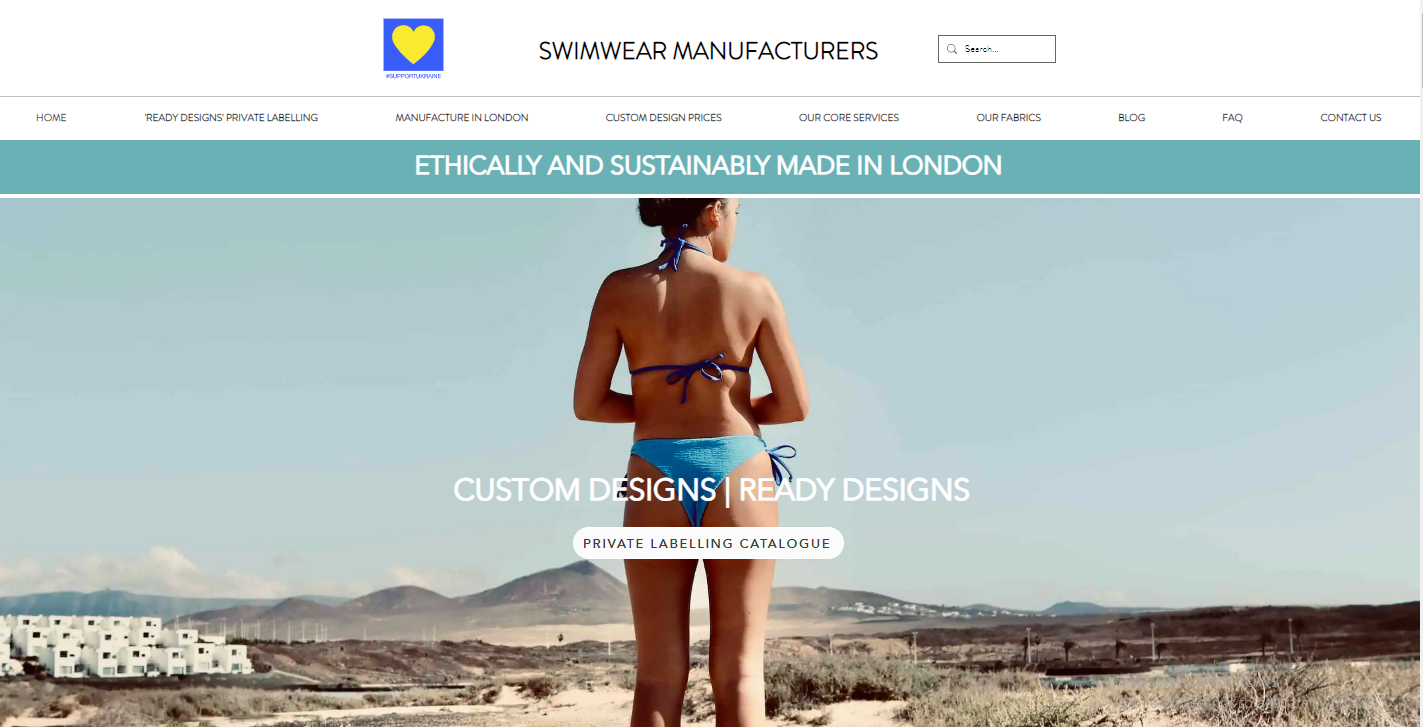The image captures a screenshot of a website with a clean, white header. At the top, the heading "Swimwear Manufacturers" stands prominently in black text on a white background. To the left of this heading is a blue square with a yellow heart inside, while a black rectangle on the right appears to contain text that is too small to read clearly. Below this header, there are nine navigation tabs, starting with "Home" and followed by "Reach Designs," "Private Labeling," "Manufacture in London," "Custom Design Prices," "Our Core Services," "Our Fabrics," "Blog," "FAQ," and "Contact Us." Beneath these tabs is a turquoise bar with the phrase "Ethically and Sustainably Made in London" in white text.

The main section of the webpage features a color photograph of a young woman seen from behind, standing in what looks like a desert area with dry shrubbery and light brown ground. She is wearing a blue bikini and facing away from the camera, showcasing the straps of her swimwear. To the left of the woman, there appears to be a village with white buildings situated on a hill, resembling architecture one might find in Greece or the Middle East. The horizon is marked by low mountains and a sky with a greenish-blue hue, accented by clouds along the left side. The bright sunlight casts shadows on the woman's back, adding to the visual interest of the image. The webpage layout, combined with the photograph, creates a striking and informative presentation for the "Swimwear Manufacturers" site.